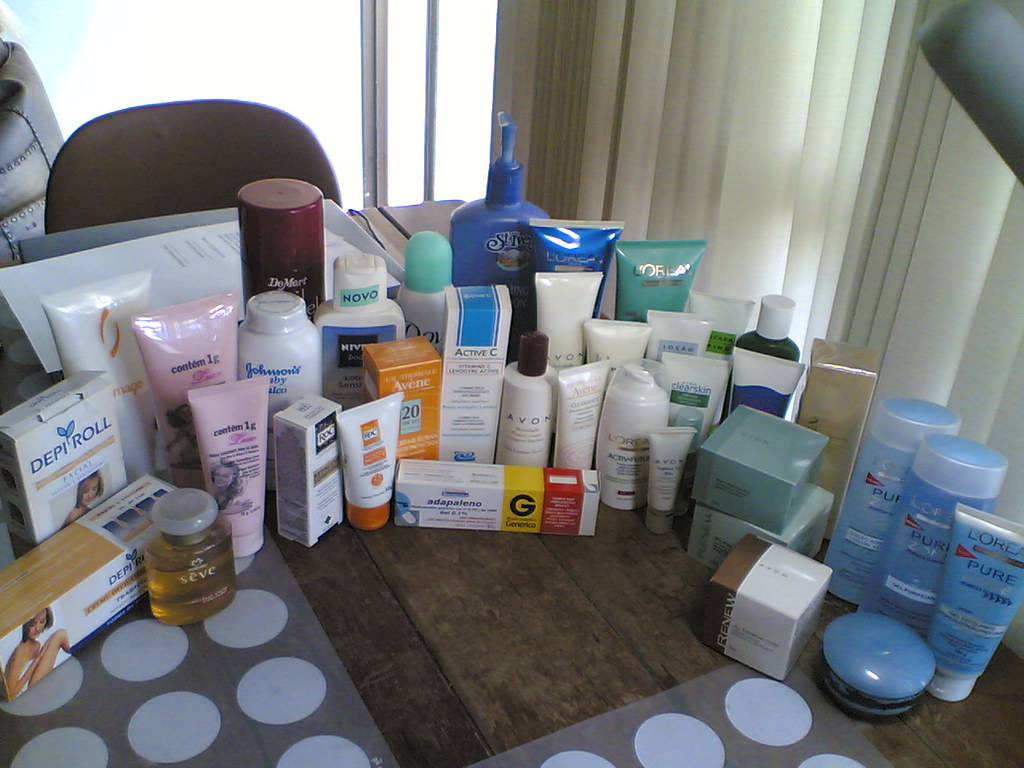This color photograph features a table with a medium brown hardwood surface. On the right side of the image, white vertical blinds partially cover a window, and in the upper left-hand corner, a portion of the open window, where there are no blinds, is visible. Sitting on the table is an extensive assortment of cosmetic and skincare products. Most of these items are contained in plastic tubes that stand upright with their caps positioned at the bottom. 

In the bottom right-hand corner of the table, there's a turquoise blue product from L'Oreal. Adjacent to it, there are two additional plastic bottles of a similar blue hue, also presumably from L'Oreal. Moving towards the left, there are a couple of boxes which are likely filled with cosmetics. One box is light green, positioned above a white box, while another box combines brown and beige colors.

Continuing leftward, more skincare products come into view. Many are housed in either plastic bottles or tubes. Among them is a white bottle labeled "Johnson's," probably containing Johnson & Johnson’s baby powder. Towards the back of the collection, there is a large blue bottle featuring a pump handle, likely a Nivea product given its signature color. On the far left side, there are a few pink tubes, though their labels are too small to read clearly.